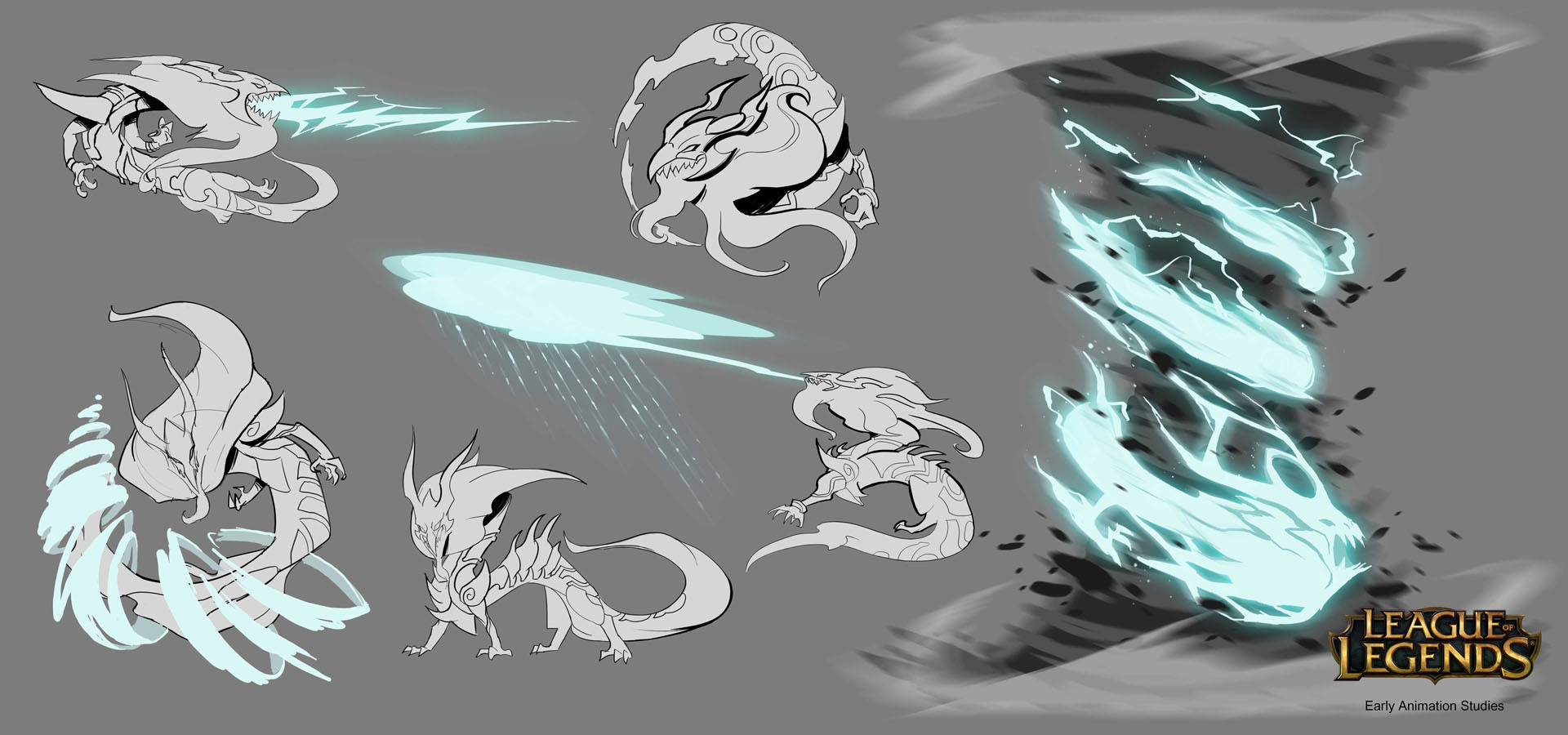This is a color illustration titled "League of Legends: Early Animation Studies" as noted in gold, capital letters at the bottom right corner on a black background. The image predominantly features gray and white tones, punctuated with light blue highlights. It showcases five different poses of a dragon-like creature with two long horns and a bird-like mask, rendered in white line drawings. These creatures are situated on various parts of the image, with two on the top and three on the bottom, appearing to perform different weather-related actions. One of them can be seen shooting lightning bolts, while another expels a light blue cloud that rains down water. Additionally, the illustration includes a dark gray tornado with a turquoise light swirled into it, located on the right side of the image, suggesting that these dragons can conjure various elemental attacks like lightning and rain. The entire composition is set against a light gray background, reinforcing the dynamic and weather-manipulating abilities of the dragon creatures.